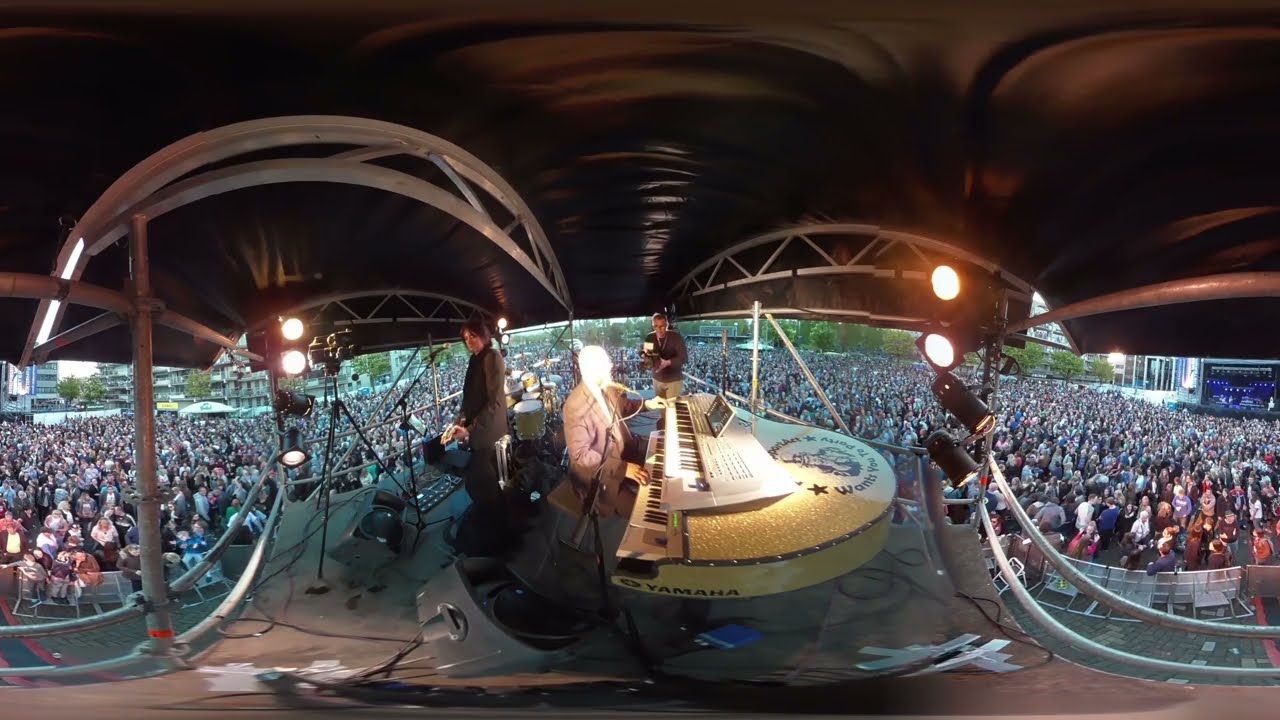This is a color photograph capturing the energy and intensity of a live concert. The main focus is a musician playing a large, two-tiered keyboard setup that combines a synthesizer and an electric piano, both of which feature black and white keys. The piano has a brown wooden body mimicking a grand piano, with sparkling gold detailing and "Yamaha" written on the side in black letters. The musician, dressed in a gray suit, is singing into a silver microphone while spotlighted.

To the left, a guitarist clad in an entirely black outfit is also singing into a silver microphone with a black base. Behind the keyboardist, a person in a gray shirt and white pants, possibly a cameraman, is seen holding a black camera. There's also a drummer with a gold, sparkly drum set matching the piano's aesthetic, although the drummer's attire is not clearly visible.

The stage itself features silver support structures, and the ceiling is a dark, almost chocolate brown, with curving architectural lines. The floor is dark gray or black, and there is a mixture of blue and silver equipment scattered about. In the background, white apartment buildings with black trim and green trees are noticeable, indicating that the venue is outdoors. 

The crowd, which numbers in the thousands, is densely packed, with attendees wearing a vibrant mix of clothing colors like blue, pink, red, and purple. The image has a highly distorted appearance, likely due to the wide-angle lens used, making the stage and audience appear stretched and curved. Nonetheless, the photo captures the vibrant atmosphere of a concert with elaborate lighting and enthusiastic fans clad in diverse, colorful attire.